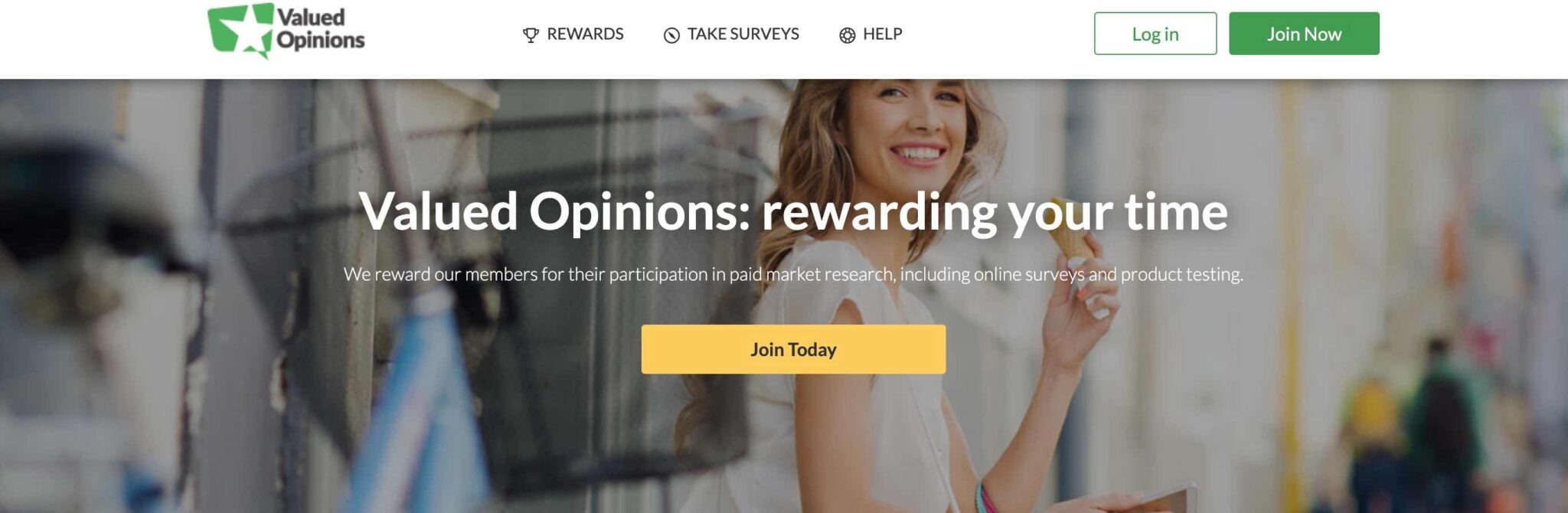Screenshot of a Website

The screenshot captures the top portion of a website. Dominating the image, there is a graphic of a slender white woman with shoulder-length blonde hair, smiling broadly while holding a pickle near her mouth. She is seated outdoors, and only her upper torso and head are visible. She has white teeth and appears to be enjoying her snack.

At the very top of the screenshot, there is a white navigation bar with several elements. On the left, a green square icon with a white five-pointed star is displayed, accompanied by black text reading "Valued Opinions." Following this, the text "Rewards" is shown alongside a small trophy icon. Next, "Take Surveys" is displayed with a clock icon, followed by a gear icon with the text "Help." 

To the right of these elements, there are two buttons. The white button reads "Log In" in green font, and the green button beside it reads "Join Now" in white font.

Beneath the navigation bar, the prominent graphic of the smiling woman with the pickle is shown. Overlaid on the image in white font are the words "Valued Opinions Rewarding Your Time. We reward our members for participating in paid market research, including online surveys and product testing." Below this text, a yellow button with black font invites users to "Join Today."